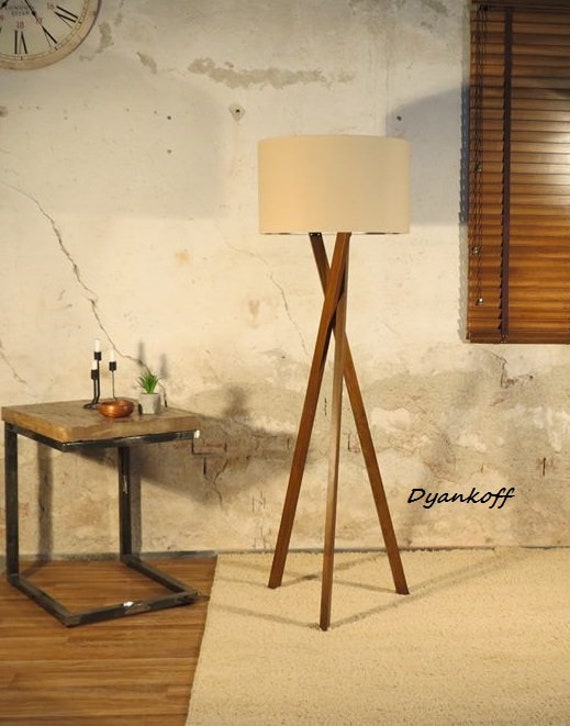The image is a highly detailed, hyper-realistic painting of a room with a blend of neutral tones and textures. The left side reveals a cracked white plaster wall, transitioning into a main area with a wooden floor that shifts into an off-white rug. Dominating the scene is an intricate lamp with glossy wooden tripod legs that crisscross two-thirds up, supporting a cylindrical beige lampshade. Below the lamp, the floor changes from wood to a beige carpet. On the wooden floor to the left sits a table with a black metal frame and a wooden top, adorned with a few items: a black metal candelabra holding three short white candles, a small green plant in a white planter, and a little copper bowl. The upper left corner features a clock, partially visible, with black Roman numerals. To the far right, there are brown wooden shutters with a black ribbon hanging beside them. On the cracked gray wall behind, you can make out a black ink signature, "D-Y-A-N-K-O-F-F," presumably the artist's. The color palette remains mostly neutral, except for the small bursts of green from the plant.